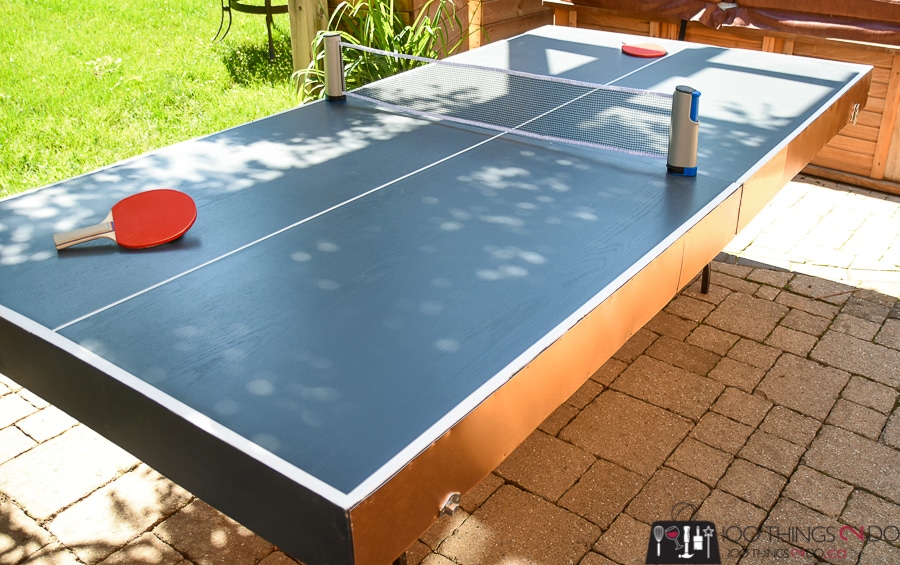This photograph depicts an outdoor ping pong table set on a stone-paved patio with a verdant lawn in the background. The scene captures the table on a covered veranda, illuminated by natural light filtering through the open side. The table itself is notably thick and built from wood, featuring a dark blue surface marked with white lines. A net, held up by two wooden posts—one curiously not positioned at the end—is stretched across the middle. Two red rubber-covered paddles lie waiting on either side of the table, suggesting a game in readiness. In the background, an outdoor kitchen setup with wooden cabinets is partially visible, adding a touch of functionality to the recreational space. A plant is also visible by the lush lawn, enhancing the tranquil ambiance of this well-curated outdoor area.